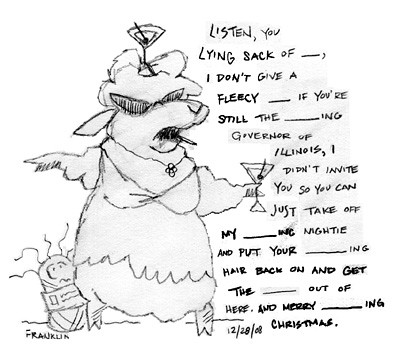The image is a hand-drawn illustration featuring a sheep dressed as a woman. The sheep, which has a humanoid appearance, is wearing a dress with ruffles at the bottom, straps resembling a bra, and a necklace with a cross. Atop its head is a martini glass with an olive and a toothpick, and it holds another martini glass with an olive in its hand. Dark cat-eye sunglasses adorn its face, and a cigarette dangles from its mouth. Adjacent to the sheep, at the bottom left, is a small, oval-shaped child figure with stringy hair holding onto the sheep’s leg, and beneath this is the signature "Franklin."

To the right of the sheep, there is a series of handwritten words in black ink. The text begins with "listen you lying sack of underscore," and continues with a series of censored statements: "I don't give a fleecy underscore if you're still the underscore ink governor of Illinois. I didn't invite you so you can just take off my underscore ink nightie and put your underscoring hair back on and get the underscore out of hair and merry underscore ink christmas 12 slash 28 slash 08." The whole scene, including the background, is colored in a dusty light blue hue.